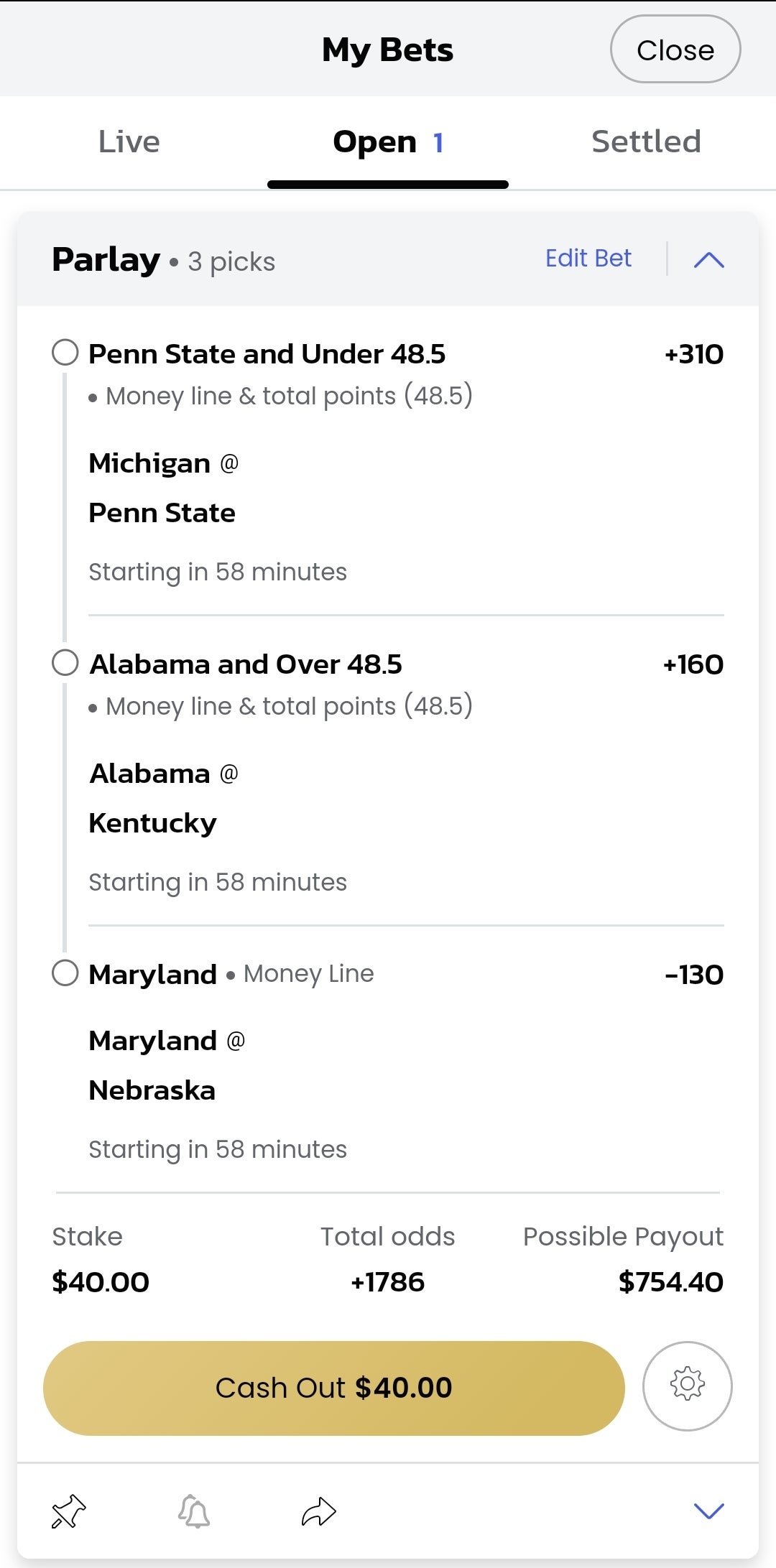Here's a cleaned-up and detailed caption for the image:

---

At the top of the screen, there's a gray header displaying betting options. The various tabs include "Live," "Open," "Settled," and "Parlay." Below, there’s a section labeled "My Bets," highlighting different active wagers and details. 

One bet is on Penn State with a spread of +48.5 and total points set at 40.5. The current status is "close." Under "Parlay," there are three picks listed: 

1. Penn State vs. [Opponent], starting in 58 minutes, with a moneyline and total points of +310 and 40.5 respectively.
2. Alabama vs. Kentucky, starting in 58 minutes, with over 40.5 total points and a moneyline of +160.
3. Maryland vs. Nebraska, starting in 58 minutes, with a Maryland moneyline of +130.

The total wagered amount on Penn State is $40, with combined odds of +1786, leading to a possible payoff of $754. 

Additional options shown include "Edit Bet," "Cashout," and settings represented by a gear icon. There is also a pin symbol, a balance indicator, and other navigational elements.

---